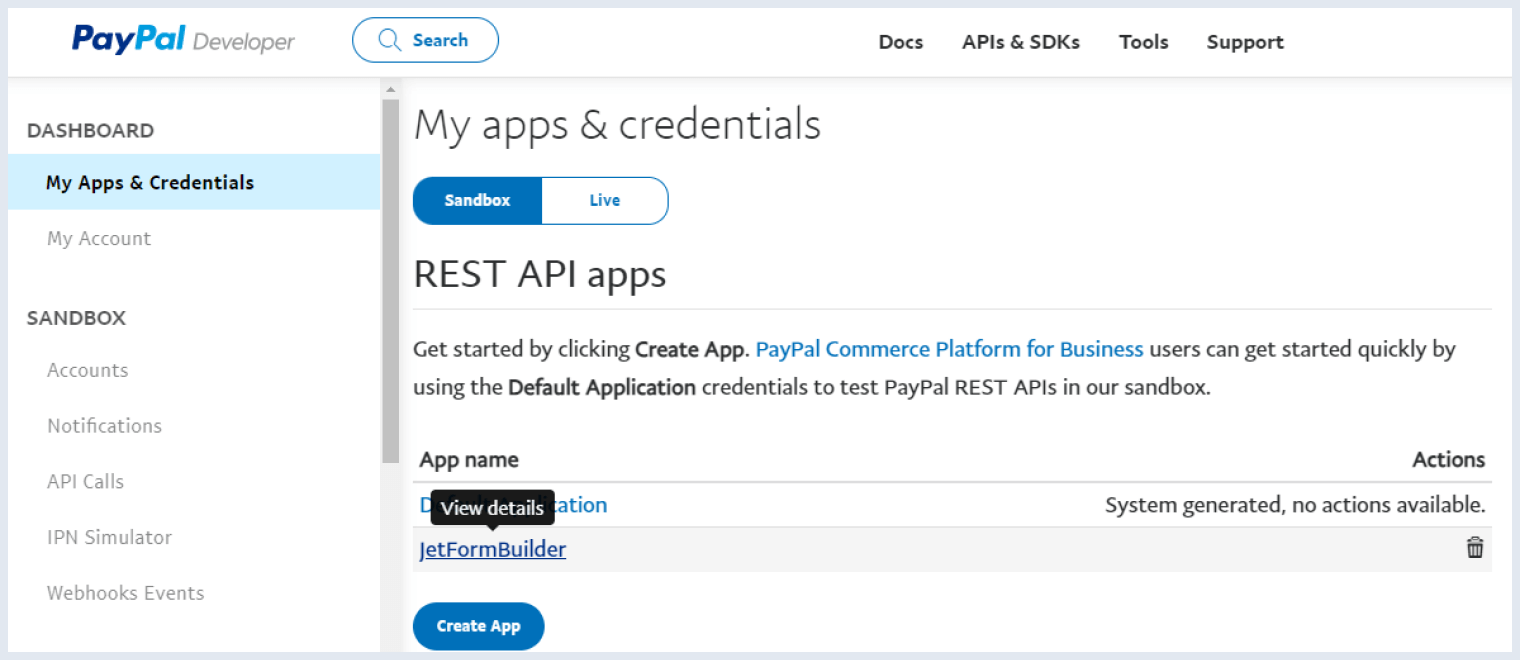The image depicts the PayPal Developer website interface. The top left corner features the "PayPal Developer" logo, with "Pay" written in dark blue, "Pal" in blue, and "Developer" in grey. To the right of the logo is a blue search button. Across the top, navigation options include "Docs," "APIs & SDKs," "Tools," and "Support."

On the left sidebar, there is a dashboard menu with several options. The highlighted option, "My Apps & Credentials," has a light blue background. Below it are additional menu items: "My Account" and "Sandbox." Under "Sandbox," the sub-menu items include "Accounts," "Notifications," "API Calls," "IBM Simulator," and "Webhooks Events."

The main section of the page, titled "My Apps & Credentials," contains two buttons: "Sandbox" in blue and "Live" in white. Beneath these buttons, a header labeled "REST API Apps" invites users to get started by clicking "Create App." The text emphasizes the "PayPal Commerce Platform for Business" in blue, explaining that users can quickly get started by using default application credentials to test PayPal REST APIs in the sandbox.

At the bottom of the main section, there is a column for "App Name" and "Actions" on the right, with a prominent blue button labeled "Create App" at the very bottom.